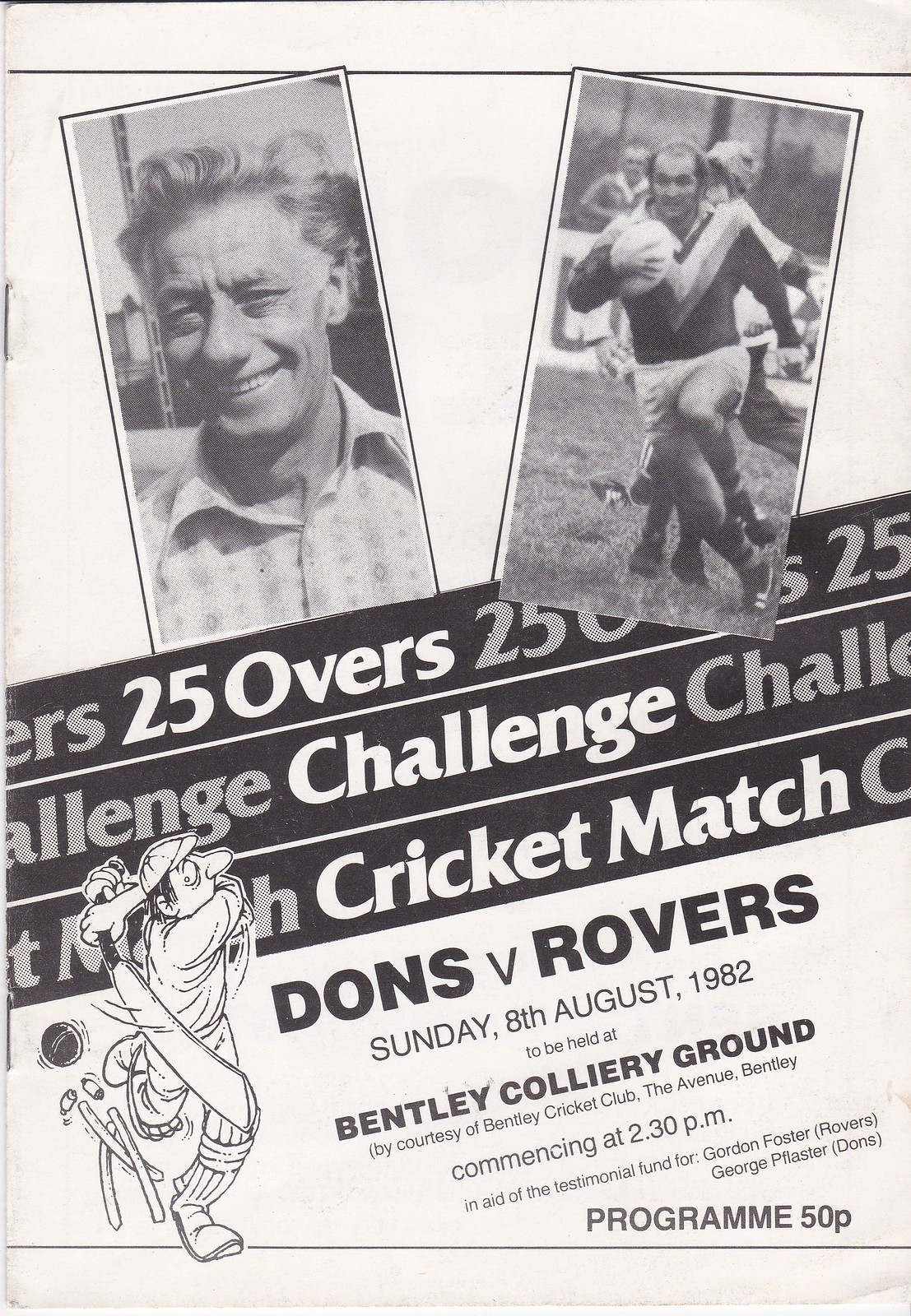The black and white cover page for a sports program features two prominent images: on the left, an older gentleman with a smile, dressed in a button-up shirt, and on the right, an action shot of a rugby player clad in a uniform, holding a white ball in his right arm. The center of the page is dominated by three diagonal red and black bands with the text "25 Overs Challenge Cricket Match." At the bottom left corner, there is a comic-style drawing of a cricket player humorously missing a ball. Adjacent to this drawing, text details the event: "Dons vs. Rovers, Sunday, 8th August 1982, to be held at Bentley Colliery Ground by courtesy of Bentley Cricket Club, The Avenue Bentley, commencing at 2.30 PM." This is followed by a note indicating it is "In aid of the testimonial fund for Gordon Foster, Rovers," and credits featuring "George Plaster, Dons." The program is priced at 50p.